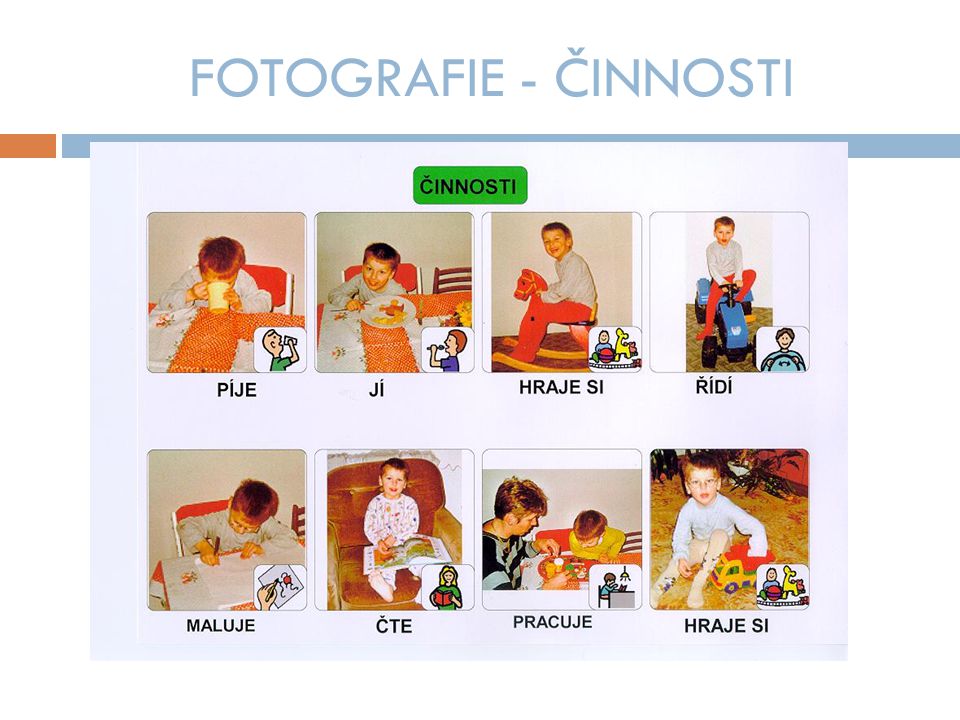The image is titled "Photography Sinosti" in light blue-gray block letters, with the accented word "Sinosti" appearing again below in a green rectangular box with rounded corners. Eight small photos of a young boy, possibly aged two or three, are arranged in two rows of four, each against a white background which overlaps a blue stripe running horizontally above the photos. The top row of photos shows the boy engaged in various activities: seated at a table with a yellow cup in front of him, looking at a plate of food, riding a rocking horse, and sitting on a blue toy tractor. Below each photo is a caption in black, possibly denoting the action being performed. The second row features the boy drawing at a table, sitting in a brown leather chair with a book, sitting at a table with a woman beside him, and playing with a yellow toy car on the floor. Each image is accompanied by a small cartoon icon in the lower right corner depicting the respective activity. The photos collectively depict the child's playful and interactive moments, capturing a range of expressions and actions.